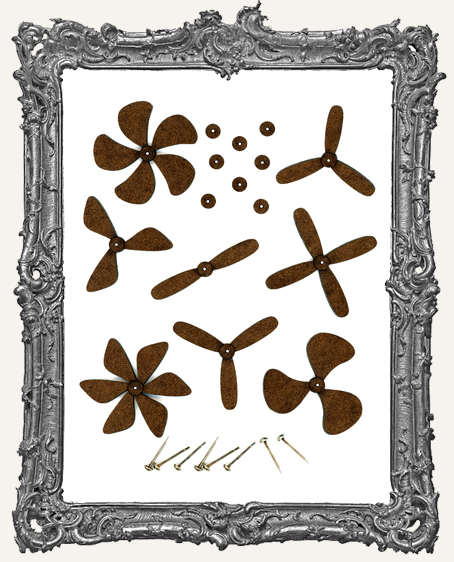The photograph showcases a beautifully detailed color image anchored by an intricate silver frame adorned with floral and vine-like engravings. Inside the frame, there's an array of meticulously carved wooden propellers, showcasing a fascinating collection of various designs and blade counts, prominently ranging from two to six blades. The majority of the propellers feature three blades, though there are notable exceptions with two, four, and a rare six-blade design. Accompanying these propellers are additional components, such as washers and pins, arranged thoughtfully in the display. The propellers’ rich brown hues contrast elegantly with their silver accents, creating a visually striking focus. Positioned within the frame, the different propellers vary in thickness and form, with some appearing more suited for maritime use while others suggest aviation purposes, particularly in model airplanes. The overall layout and diverse assortment reflect a careful curation, making it an intriguing and aesthetically pleasing piece of art that could adorn a wall or grace a desk.